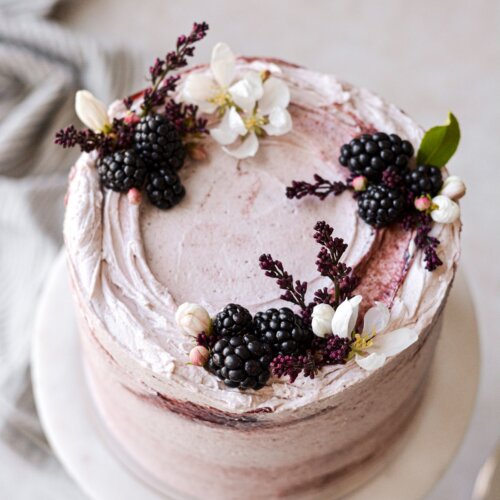This image depicts an elegantly styled, approximately six-inch circular cake adorned with blackberries, delicate white flowers with yellow centers, and green leaves, complemented by sprigs of a purple flower. The cake is frosted in a blend of pink and white, applied in a rustic, natural manner, giving it an organic appearance with colors blending smoothly together. Photographed from above, the cake is set centrally against a soft, blurry background that appears to be a rumpled white or gray and white striped tablecloth, emphasizing the cake's details. The frosting on the cake's top forms a thicker, swirled rim, adding texture and depth where the blackberries, flowers, and decorative elements are strategically placed, creating an elegant and appealing look.